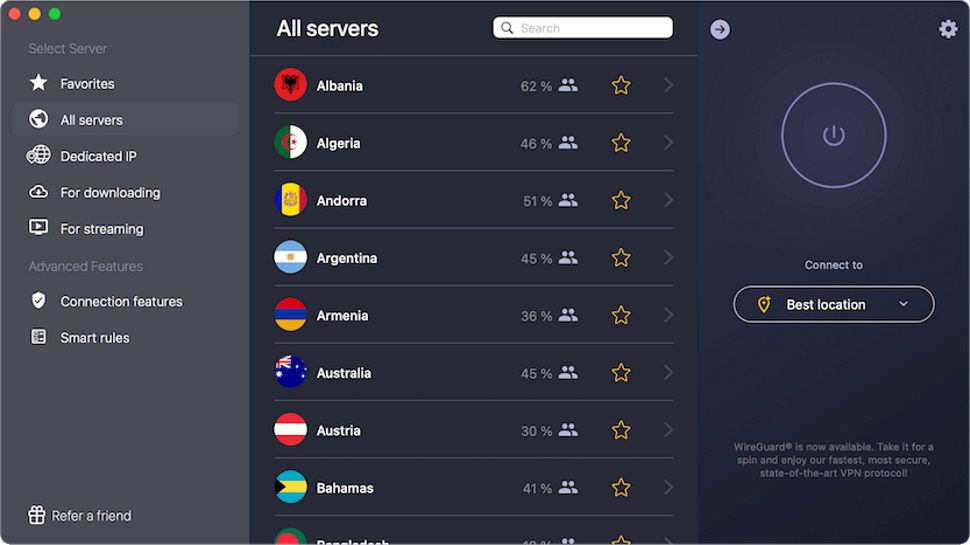Screenshot of a Mac Computer Displaying a Server List

This image is a screenshot of a server list, captured from a Mac computer screen. The screenshot is wider than it is tall and depicts a sleek black window with rounded corners. In the upper left-hand corner of this window, the familiar red, yellow, and green circles characteristic of Mac OS windows are visible.

On the left side of the window, a lighter gray toolbar is present. At the top of the toolbar, the text "Select Server" is displayed. Below this heading, there are various selectable categories, each accompanied by a specific icon. These categories include "Favorites" (marked with a star icon), "All Servers," "Dedicated IP," "For Downloading," and "For Streaming." Further down, there is a section labeled "Advanced Features," which encompasses "Connection Features" and "Smart Rules." The toolbar concludes with a "Refer a Friend" option at the bottom.

On the right side of the window, the text "All Servers" appears in white font at the top left corner. Centrally located within the main area is a search bar, although the servers are currently listed by country in alphabetical order. The visible countries include Albania, Algeria, Andorra, Argentina, Armenia, Australia, Austria, and the Bahamas. Each country name is paired with a circular icon displaying its national flag to the left, followed by a percentage indicating the current server usage (e.g., Albania 62%, Bahamas 41%). To the right of these percentages, there are gold star icons, which likely serve as an option to mark the servers as favorites.

Additionally, there is another smaller window or panel on the right-hand side of the main window, which contains various buttons, although their specific functions are not detailed in the screenshot.